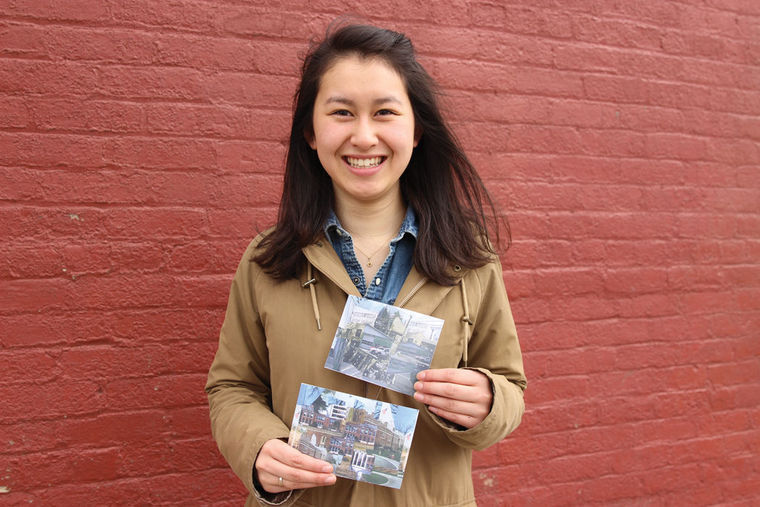In front of a red brick wall, a young woman who appears to be in her twenties is standing and smiling brightly. She has black hair that falls slightly past her shoulders, with one side pulled back, and her hair is gently blowing, suggesting a slightly windy day. She has dark eyes and pink lips, revealing a set of white teeth in her smile. She's wearing a blue denim shirt with a collar underneath a brown jacket that features tan drawstrings and a hood. Around her neck, she sports a gold necklace that peeks out from under her coat. On her right hand, she wears a silver ring. She is holding up two black and white pictures, one on top of the other, with her left hand. The picture on top shows a house, a car, and blue skies, while the bottom picture depicts a red building with cars and a blue sky.